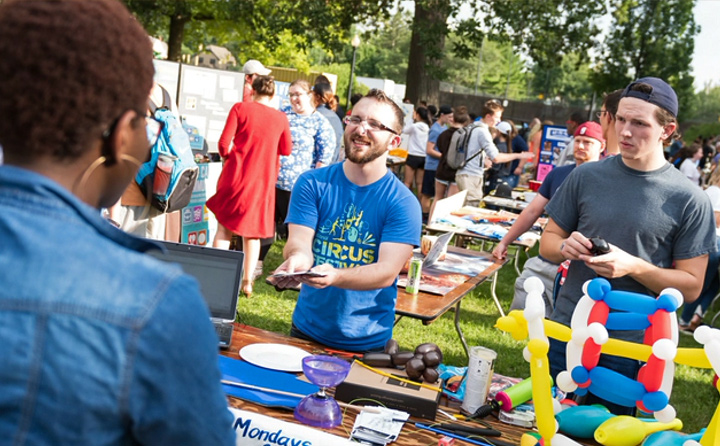The photograph depicts a lively game fair set in a lush garden adorned with tall, green trees. Several wooden folding tables are arranged throughout the area, displaying a variety of colorful items such as drawings, bags, and small toys, including balloon animals. In the foreground, on the left side, stands an African American woman with short brown curly hair, dressed in a blue denim dress and wearing large hoop earrings. She is engaging in a transaction with a man to her right, who is holding up some money and smiling. This man wears glasses, has a short beard, and dons a blue crew neck shirt with a gold graphic.

Next to them, another man, who appears somewhat impatient, holds a black, round object. He is dressed in a charcoal short-sleeve t-shirt, a backwards baseball cap, and is looking up towards the woman. On the table in front of them are various items including a purple funnel, black cylindrical shapes, a jar filled with change, a cash register, a calculating device, and several colorful balloon figures. Further in the background, more people can be seen mingling around the tables, with the fairgrounds bordered by a fence and dark green trees towering above, encapsulating the spirited atmosphere of the outdoor event.